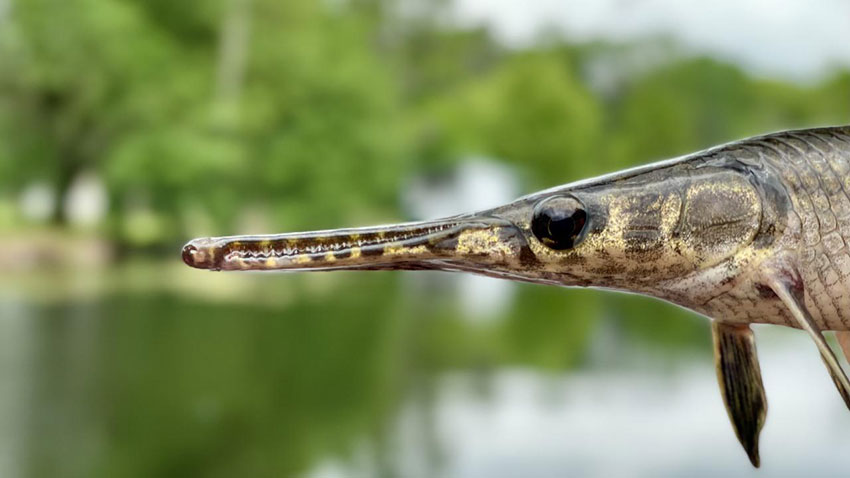This close-up photograph captures a highly detailed and photorealistic side view of a fish, possibly a type of gar, held just above a serene lake. The fish, mostly brown with gold accents and some mottled spots on its head, is showcased against an out-of-focus background of green water reflecting a tree-lined shore. The fish is oriented with its long, slender, and serrated alligator-like snout pointing towards the left, showcasing tiny, sharp teeth. Its large black eye and pectoral fins are prominently visible, with the fins hanging downwards. Part of a finger holding the fish is visible on the right edge of the image. The shimmering scales and textures of the fish are captured in high detail, adding to the lifelike quality of the photograph.